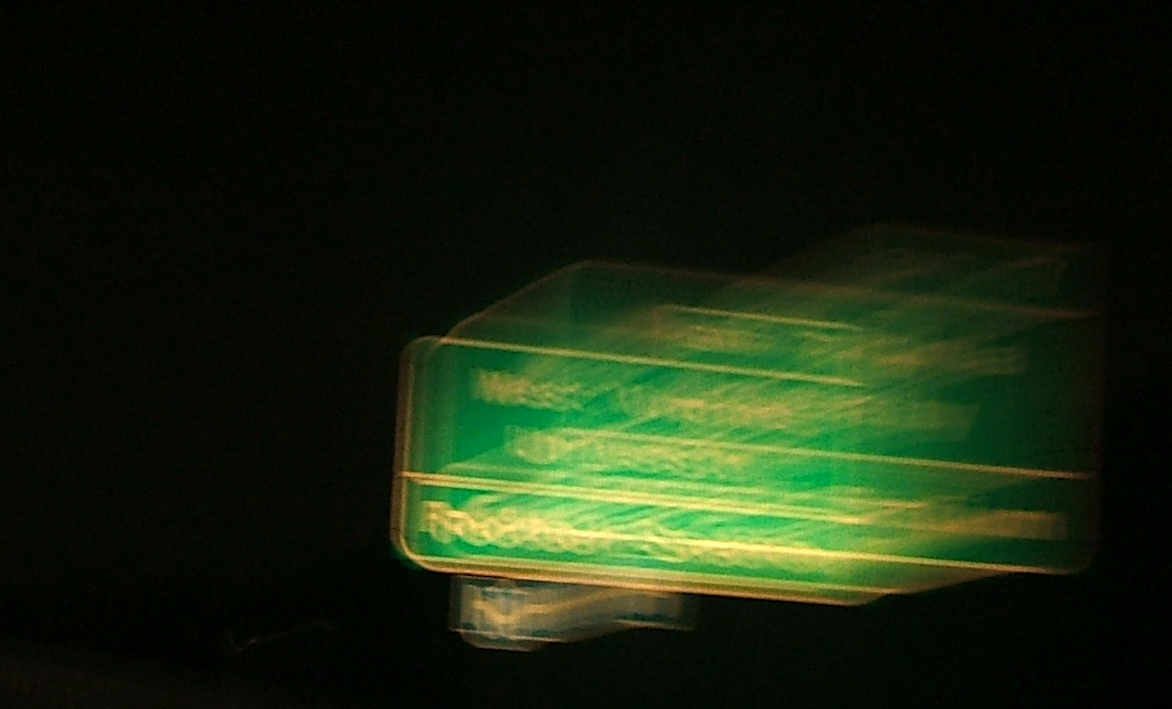This photograph captures a freeway sign set against a pitch-black night sky. The sign itself appears green with distinct white lettering, though the image is notably blurry and out of focus, suggesting it was taken swiftly, possibly while moving. The legible text includes the word "West," situated in the top section of the sign. There are additional lines of text below, but their details remain indiscernible due to the lack of clarity. An overhead light faintly illuminates the sign, emphasizing its contours despite the overall obscurity. The photo effectively conveys the urgency and motion associated with its capture.